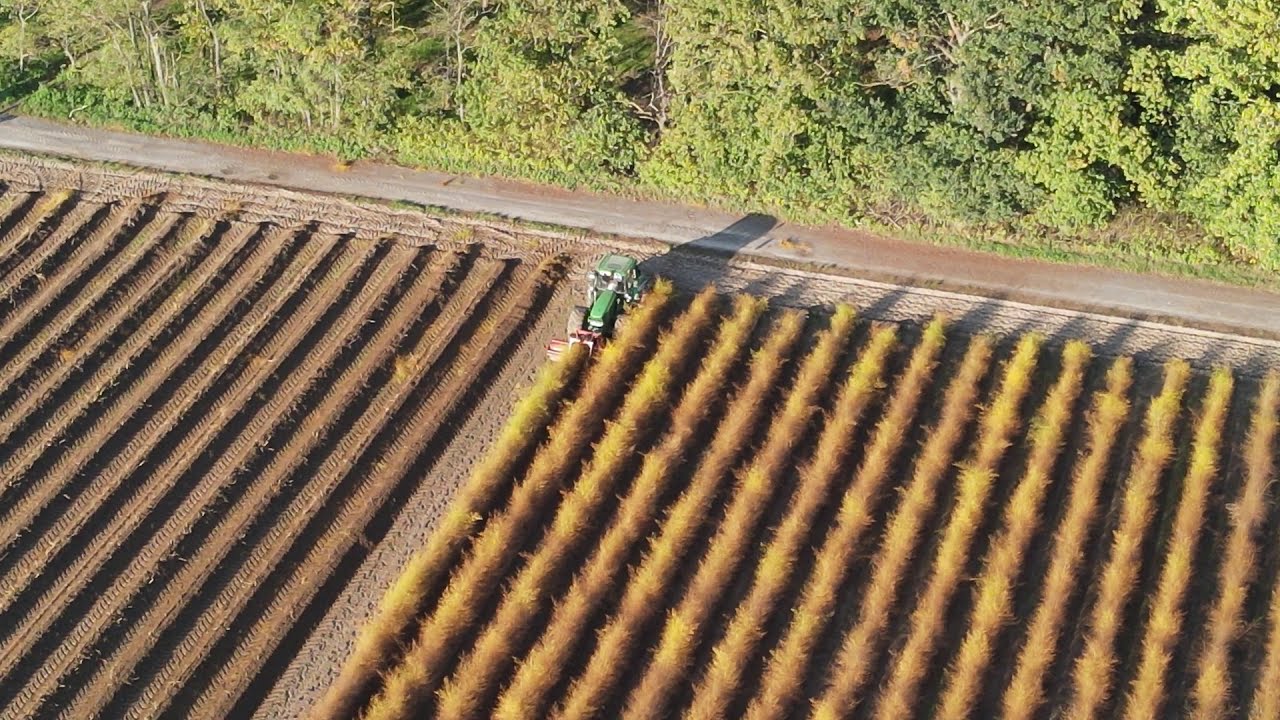This aerial landscape photograph captures an agricultural land plot in vivid detail. Rows of plants, featuring autumnal shades of brown, yellow, and gold, spread across the field. A dark green tractor, centrally positioned, moves diagonally from the back right towards the front left, actively plowing one of the rows. Evidence of its progress is seen in the cleared rows of dirt trailing behind it. The plot showcases about 20 such rows, some already cultivated and others awaiting attention. Beyond the field lies a horizontally oriented dirt road that separates the farmland from a lush, bushy area full of trees, shrubs, and grasses. The scene, captured from a drone, emphasizes the methodical work ongoing in this rural farm setting, combining the raw elements of nature with human agricultural activity.